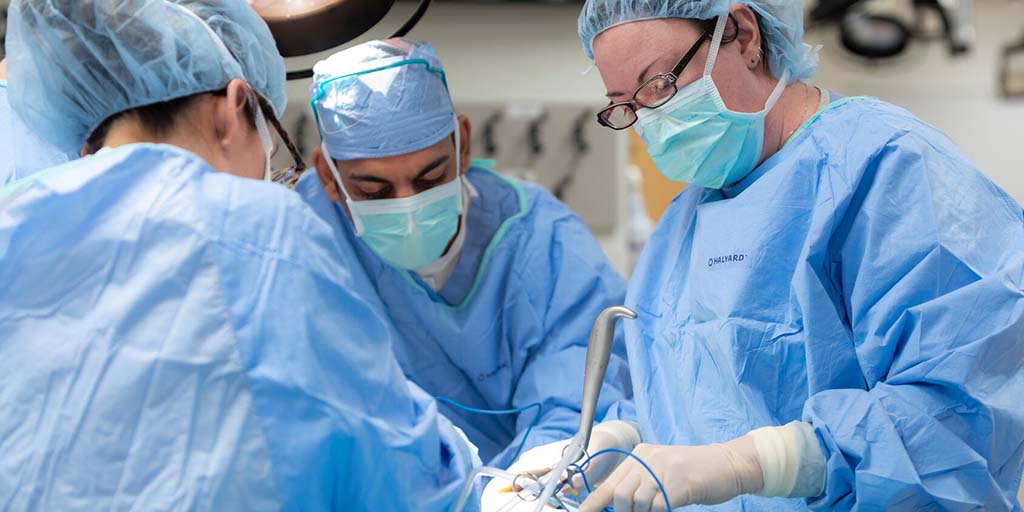The image is a detailed color photograph in landscape orientation depicting a trio of medical professionals, likely surgeons, engaged in a procedure in an operating room. All three are clad in blue surgical caps, masks, and gowns, symbolizing a sterile environment. The woman on the right, identifiable by her black glasses and the name tag 'O.H.A.D.A.R.D.' on her chest, is intently focused on her task. She is wearing white vinyl gloves and manipulating a silver metallic tool with a vertical handle, possibly looping strings around it. The male surgeon in the middle is also absorbed in the procedure, while the third individual, another woman positioned on the far left, is shown with her back turned to the camera. Her face is not visible, contributing to a sense of busy anonymity among the medical team. Illuminating their workspace is an overhead light, casting a focus on their meticulous work. The background, slightly out of focus, contains typical operating room equipment, enhancing the realism and authentic atmosphere of this high-stakes, medical environment.